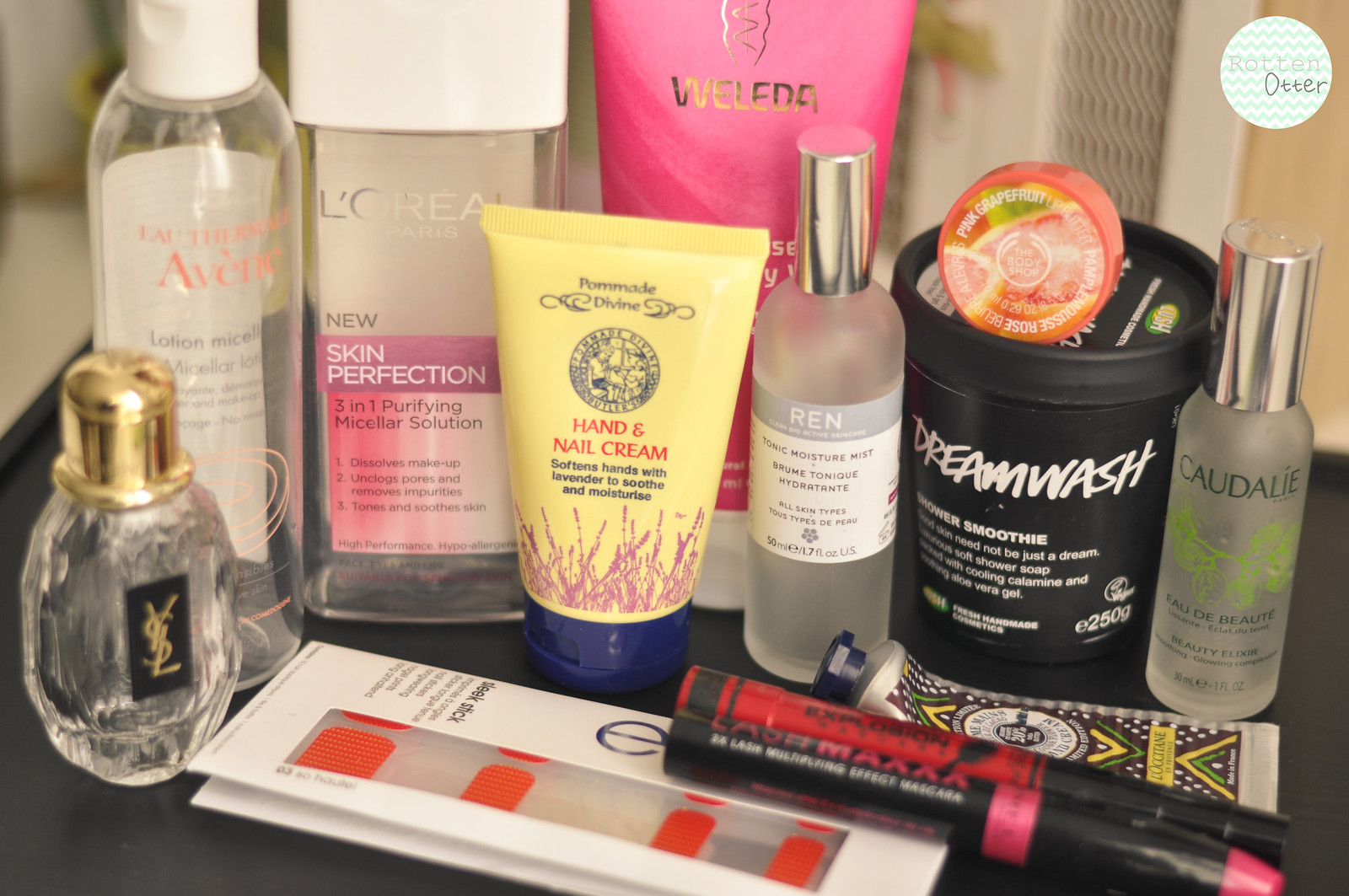A sleek black table is adorned with an array of self-care products. On the far left, a sophisticated cologne bottle features textured glass and a brass top. Behind and to its right, a towering Aveeno product stands in a transparent plastic bottle with peach-colored lettering, clearly labeled as a lotion in gray writing. Adjacent to the Aveeno is a L'Oreal Skin Perfection product, housed in a transparent container with a white cap, matching the height of the lotion bottle. In front and slightly to the right sits a tube of hand and nail cream, vibrant in a yellow container with a blue lid. Behind this is a product from Wellina, packaged in eye-catching pink plastic. To the front and right of the Wellina is an R.E.N. product, and further right, a Dreamwash product contained in a black tub. Next to this tub is a Caudalie item, elegantly presented in a frosted glass bottle with a silver top. Completing the display in front of all these items is a long, rectangular palette of eye makeup, adding a touch of beauty essentials to the self-care collection.